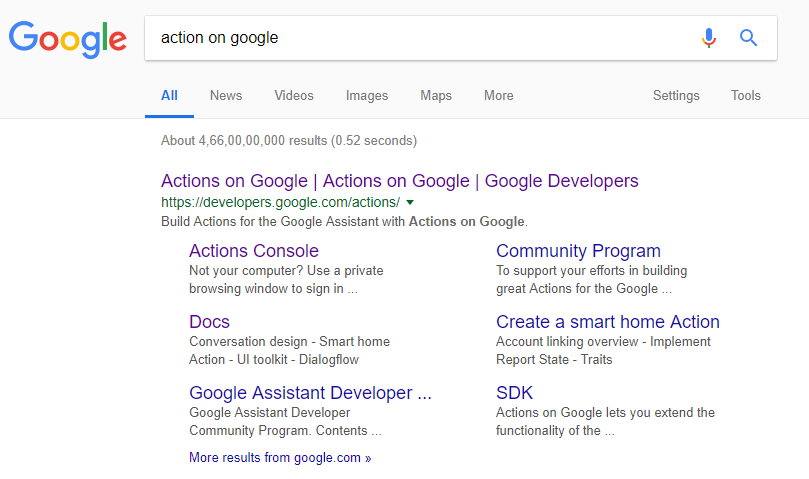This image is a detailed screenshot of a Google search results page, likely viewed on a tablet or iPad. Dominating the upper portion, the iconic Google logo is prominently displayed on the left, showcasing its recognizable color scheme: a blue "G," a red "O," a yellow "O," a blue "G," a green "L," and a red "E". Centered beneath the logo, there is a search bar containing the query "action on Google," followed by a microphone icon for voice search and a magnifying glass icon signifying the search function.

Directly below the search bar, a navigation bar offers several clickable sections including "All," "News," "Videos," "Images," "Maps," "More," "Settings," and "Tools." Following this, the search engine displays the result statistics: approximately 4.66 billion results (or possibly trillion), generated in 0.52 seconds.

The primary search result shown is for the Google Developers page related to "Actions on Google." The URL is https://developers.google.com/actions. This page includes resources like the Actions Console, Documentation, Google Assistant Developer tools, and the community program. Users can learn how to create Smart Home actions and access the Software Development Kit (SDK).